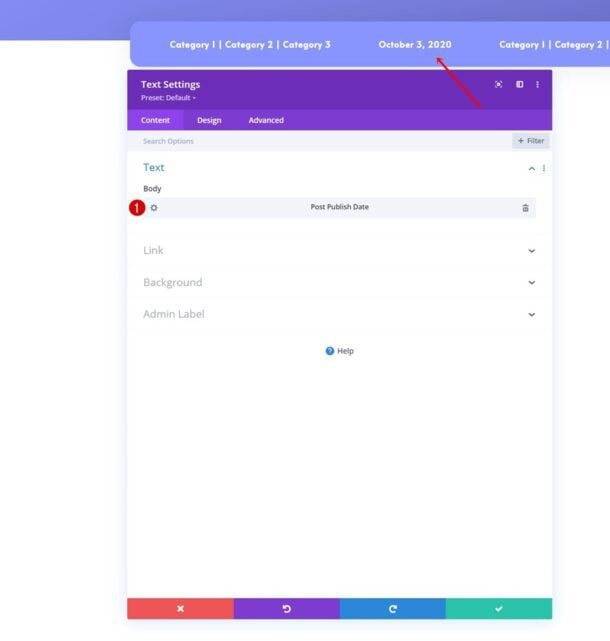In this screenshot of a web application interface, we are looking at the setup for composing a body of text, likely for sending as a message or email. At the topmost section, there is a prominent blue banner that features categories numbered 1, 2, and 3, with a date displayed to the right: October 3rd, 2020. This date is flanked again by categories 1, 2, and 3 to its right. Immediately below, there is a pop-out window designated for text settings, currently set to default.

In the upper-right corner of the interface, three icons are visible: one to display all open windows, one to minimize the current window, and one that provides access to a drop-down list. Below this set of icons are three tabs: "Content," "Design," and "Events," with the "Content" tab being actively displayed.

Further down, there are search options that enable filtering, followed by the main body text area. In this section, users can manage publishing dates, insert links, add backgrounds, and customize admin labels. Below this functionality, a help icon and link are available for additional assistance.

At the very bottom of the interface, four buttons are visible: "Undo," "Redo," a checkmark button presumably for confirmation, and one additional unmentioned button.